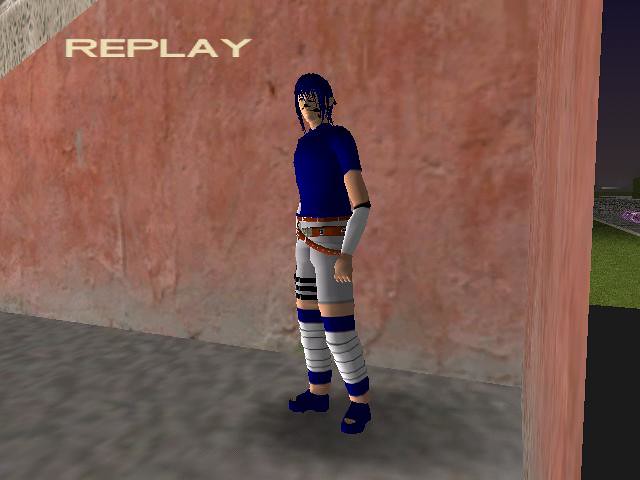The image shows a colorful scene resembling an interface from a computer game, indicated by the white text "replay" in the upper left-hand corner. Adjacent to the text is a grey corner situated on the left side. The background features a reddish wall at the top and transitions to a grey surface at the bottom. Standing on the grey surface is a player character.

The character is dressed in a distinctive outfit that includes a blue cap or helmet. The facial features of the character are obscured and appear unusual, marked by black lines that may be indicative of a game glitch. The character is wearing a short-sleeved blue top paired with grey shorts that have lines on the lower part of the right leg. A multi-colored belt is strapped around the waist.

The character’s legs are adorned with leg warmers that feature a combination of blue at the top, black stripes, grey, and blue shoes. Notably, the toe of the left shoe looks exposed, which could also be a glitch. Additionally, the character has a silver arm warmer on the lower part of its left arm, possibly another glitch.

In the lower right-hand corner of the scene, there is what appears to be the edge of a playing pitch. The pitch is green in the middle and is bordered by black at both the top and bottom sections.